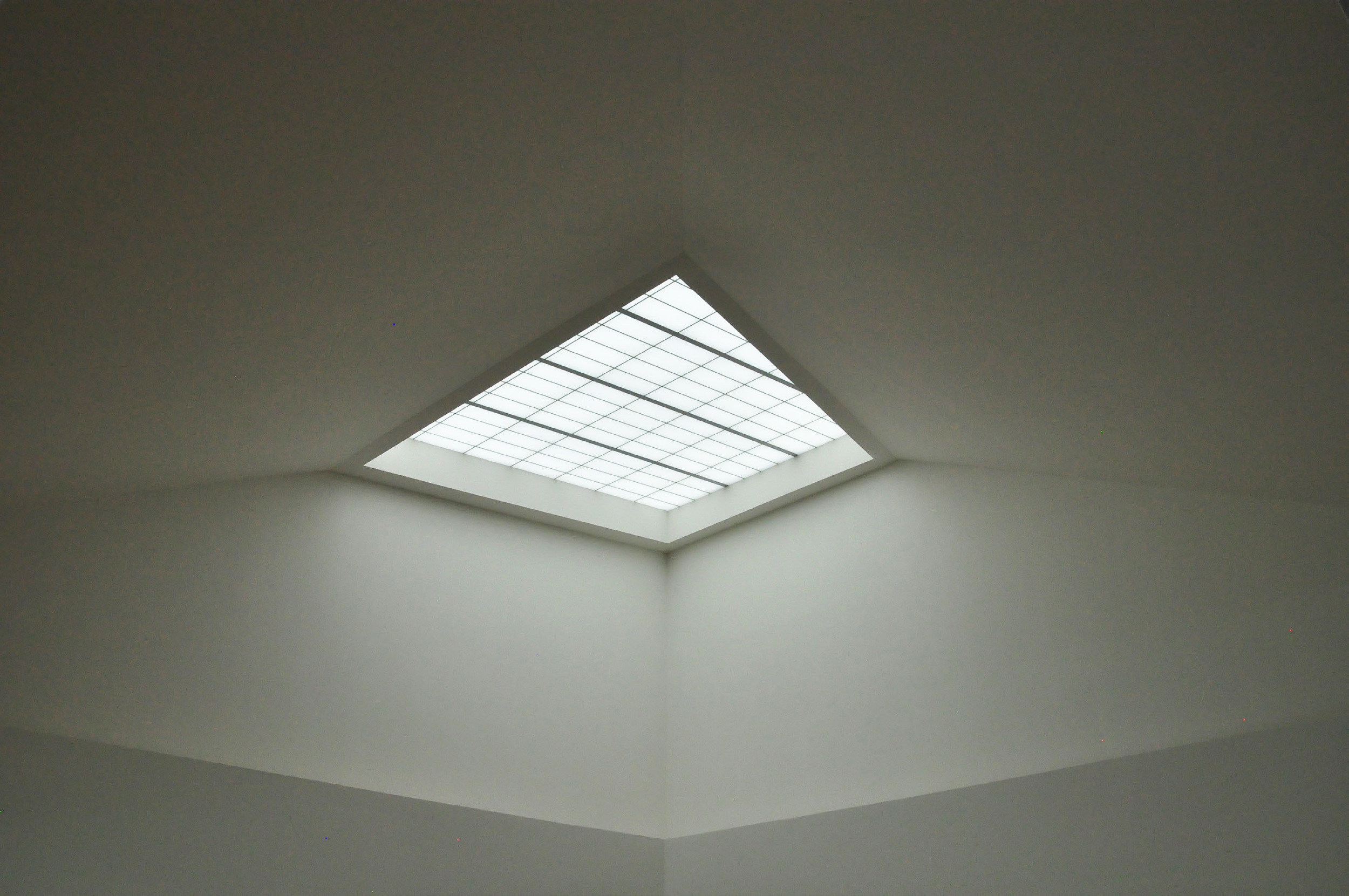This detailed photograph captures the ceiling of a room, prominently featuring a trapezoidal skylight positioned diagonally at the center. The skylight is defined by three thicker, horizontal black bars and additional smaller crosshatched bars, allowing light to project into the room. The ceiling, painted in a lighter gray, contrasts with the darker gray of the lower half of the walls. Architectural angles draw the eye upward toward the skylight, where light flows in and casts interesting shadows throughout the space. The unique slant and layout of the skylight, combined with the variation in wall colors, create a visually captivating and dynamic interior.